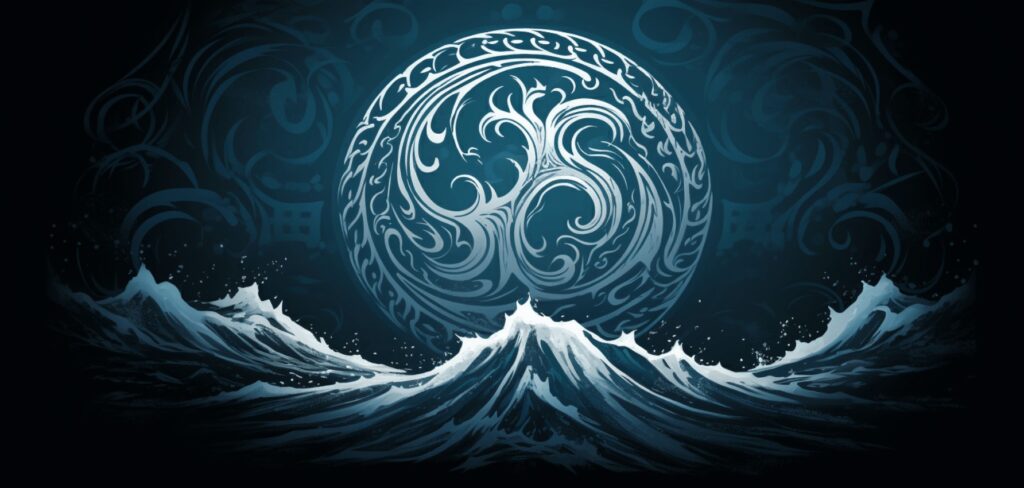This intricate computer-generated artwork features a highly stylized emblem set against a very dark blue background. At the base of the image, there's a depiction of ocean waves with pointed crests and whitecaps, portrayed in a very dark blue and white color scheme, giving the effect of a nighttime sea. Above these waves, the background is adorned with ornate, swirling flourishes that appear to create a meaningful and visually captivating pattern. Central to the piece is a large, bright white circle outlined by a design resembling an interlocking chain. Within this circle, a swirling motif expands outward, creating multiple points and adding a sense of movement and complexity. The overall composition evokes a sense of both elegance and tranquility, with the swirling lines and patterns reminiscent of royal medallions or traditional coat of arms designs.